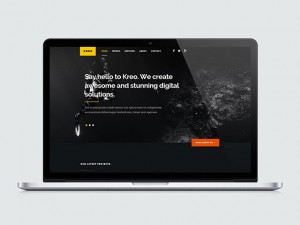The image features a sleek MacBook with a prominently displayed screen. The screen warmly greets with the words "Say Hello to Creo" and proudly declares, "We create awesome and stunning digital solutions." The overall color scheme is a combination of black, red, and silver, which are elegantly set against a clean white background. There is a noticeable light reflection or a soft light cast on the right side of the MacBook's screen, adding a dynamic touch to the visual presentation.